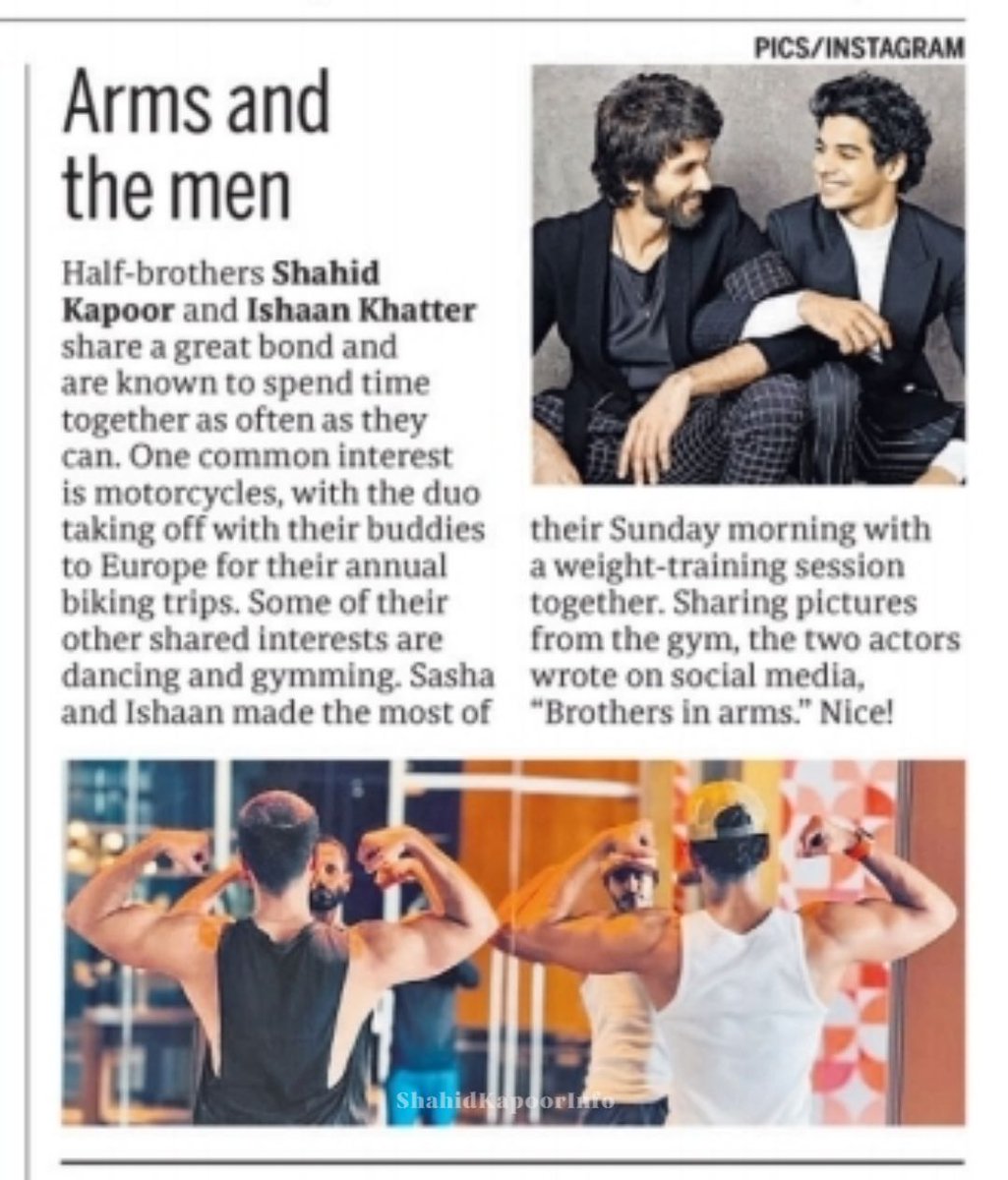The image is a scan or photograph of a newspaper article titled "Arms and the Men," set against a white background with black text. Prominently featured are half-brothers Shahid Kapoor and Ishan Khattar, who share a close bond. The top right corner features an inset color photo of the brothers, dressed in dark suits with casual shirts and dress pants, smiling at each other with their arms linked. Above this image, text reads "pics/Instagram." Throughout the article, it details their shared interests, including motorcycles, dancing, and gymming. It mentions their annual biking trips to Europe with friends. The bottom of the article includes a color photograph of the two men in a gym, facing a mirror and flexing their muscles while wearing tank tops; Shahid in a black tank top and Ishan in white. This image captures them showing off their biceps during a weight training session. The newspaper-style layout and the meticulous details highlight the brothers' camaraderie and their active lifestyle.